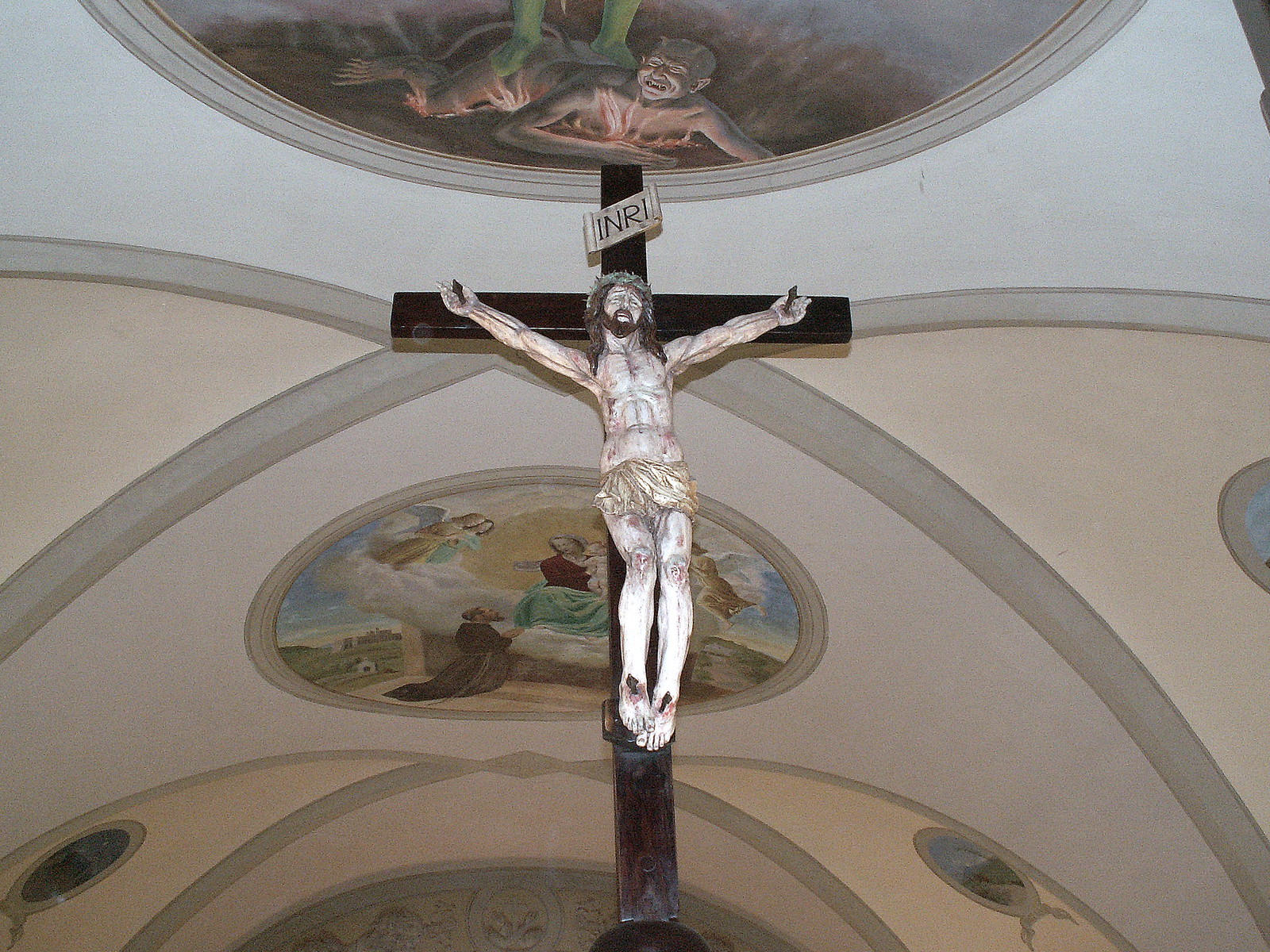The photograph captures the interior of a grand church, focusing on a prominent statue of Christ on a wooden cross, which is mounted high up near the ceiling. The statue depicts Jesus nailed to the cross through His hands and feet, exuding a profound sense of suffering. The statue is primarily white, starkly contrasting with the darker brown tones of Jesus's hair, beard, and the cross itself. Below the statue, Jesus’s feet are nailed to the vertical part of the cross.

The church's ornate ceiling arches above, richly decorated with various artworks. Directly above the statue of Christ, there is a striking illustration featuring a demon-like figure sprawled out with flames beneath it and feet pressing down on its back. This demonic figure, depicted in agony, is part of an intricate mural that includes other elements such as lines and decorative designs. Another notable part of the artwork illustrates a man in a kneeling position, potentially in prayer, accompanied by angelic figures. The interior of the church is well-lit, enhancing the visibility of these detailed and symbolic illustrations.